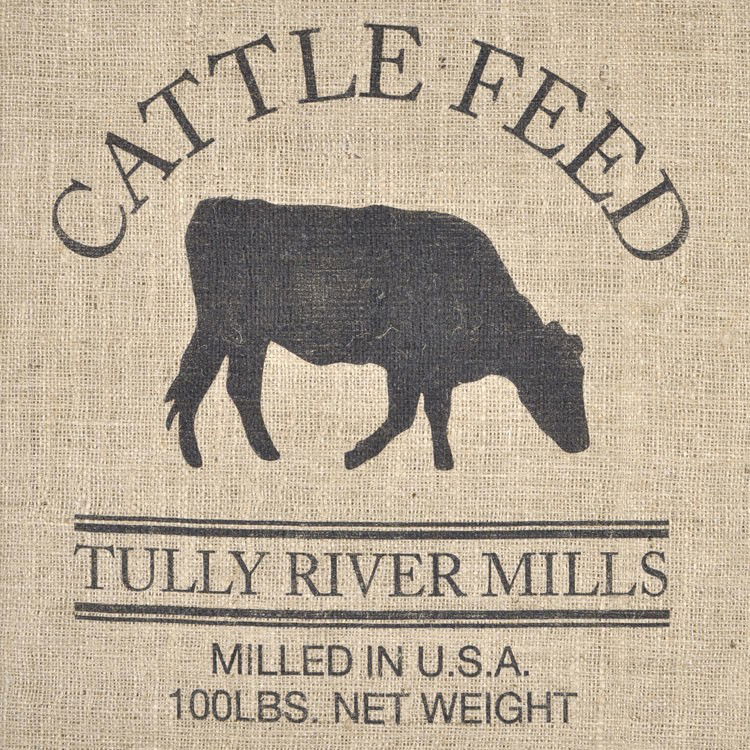This photograph captures a close-up of a tan burlap sack adorned with dark print, prominently featuring a company logo and text. Central to the image is a black silhouette of a cow, its head bent down as if grazing, with no visible tail. Above the cow, in large, arched black capital letters, the text reads "Cattlefield." Below this, inside a bordered area with lines above and below, it states "Tully River Mills," also in black capital letters but in a slightly smaller, bold font. Further below, in a more traditional, smaller font, the text "Milled in USA, 100 pounds net weight" completes the design.